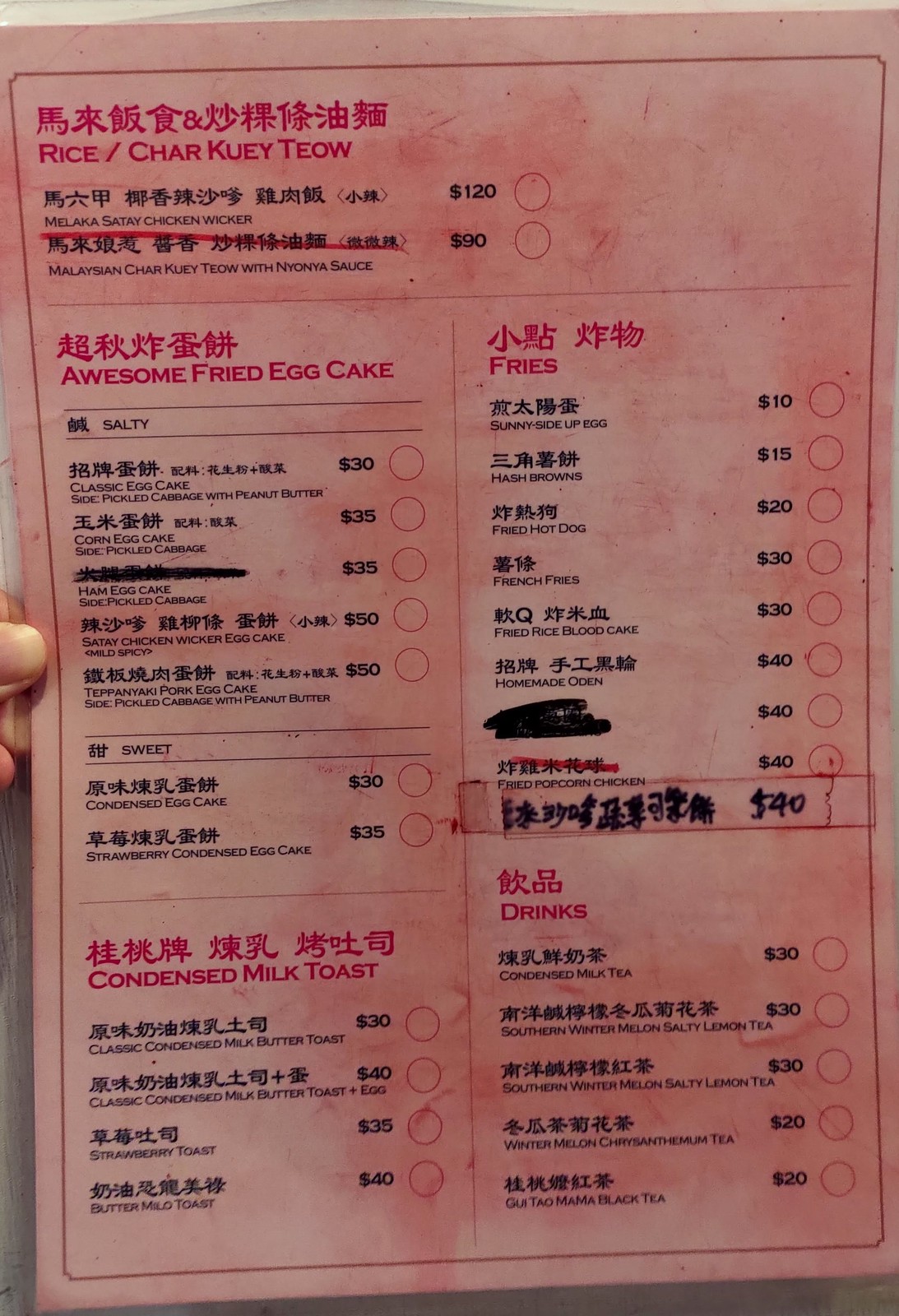This is an image of a well-used menu from a Chinese restaurant, characterized by its red tint. The top of the menu features the categories "Rice," "Char Tui," and "Tea O," with Chinese characters prominently displayed above these categories. Directly below, more Chinese characters can be seen, accompanied by the item "Me La Ga, Satay Chicken Wicker," priced at $120.

Further down, additional Chinese characters introduce "Malaysian Char Tui, Tea O with Nyona Sauce," listed for $90. Following this, there is a section in red lettering advertising "Awesome Fried Egg Cake," again accompanied by Chinese characters.

The menu then shifts to a section labeled "Salty," offering five dishes priced at $30, $35, $35, $50, and $50 respectively. Below "Salty," there is a "Sweet" section with items ranging in price from $30 to $35. The next category is "Condensed Milk Toast," featuring four items priced between $30 and $40.

On the other side of the menu, there is a section titled "Fries," which lists various dishes in both Chinese and English, with prices ranging from $10 to $40. The final category on the menu is "Drinks," offering five different types priced between $20 and $30. The overall condition of the menu suggests it has been frequently handled, adding to its red-tinted, worn appearance.